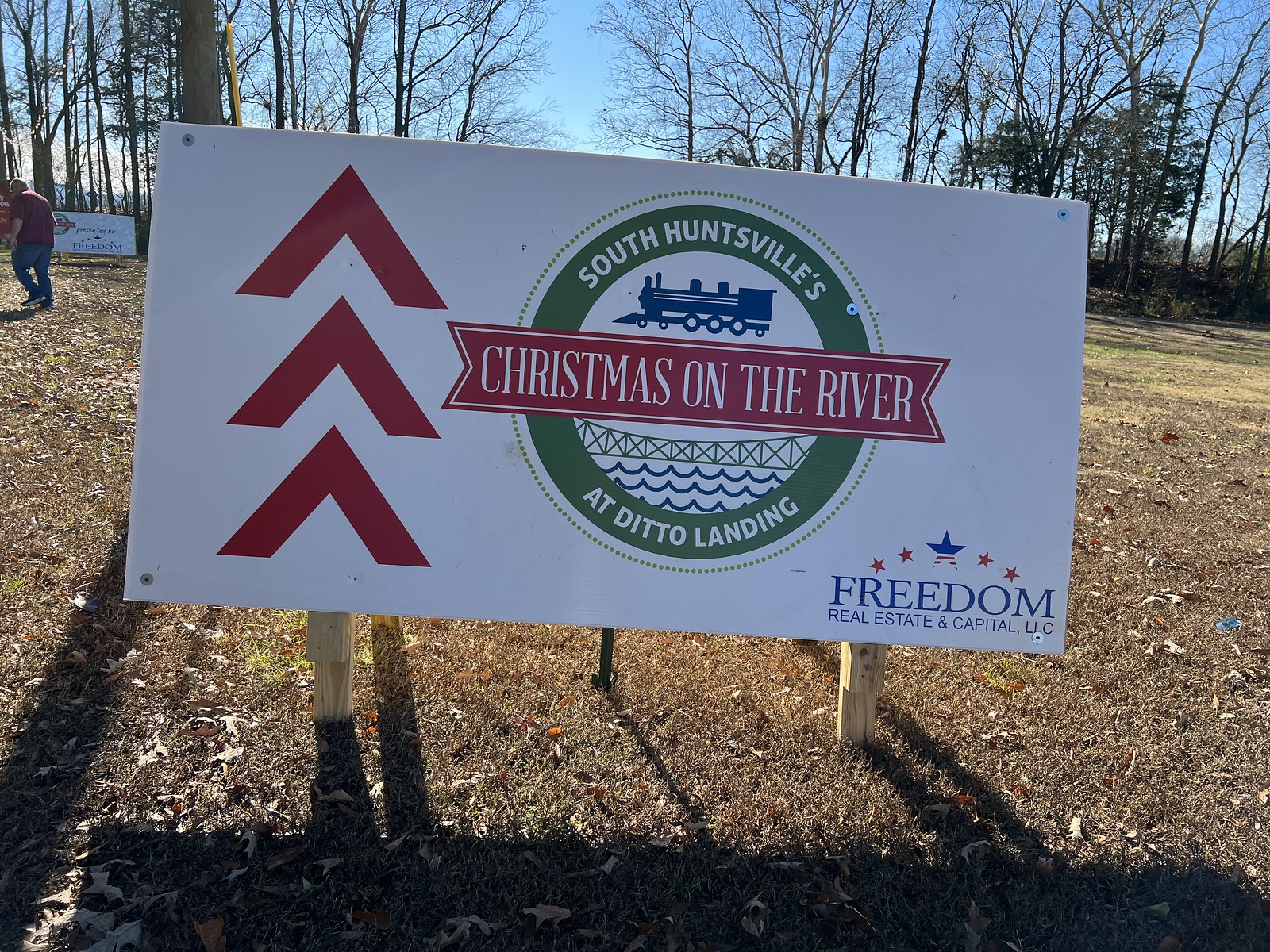The image features a large white sign firmly secured with four wooden supports, situated in a grassy clearing dotted with dead leaves. The background is filled with mostly leafless trees, a few of which retain some green foliage, beneath a clear blue sky. The sign is adorned on the left with three vertically stacked, red upward-pointing arrows. Dominating the right side of the sign is a green circular emblem. At the top of this emblem, in white text on the green background, it reads "South Huntsville," while the bottom part says "at Ditto Landing." A central ribbon across the circle proclaims "Christmas on the River." Within the emblem are icons of a train, a bridge, and blue wavy lines representing water. Additionally, the bottom right corner of the sign bears the text "Freedom Real Estate and Capital LLC." In the upper left corner of the image, a man dressed in blue jeans and a red short-sleeved shirt is seen walking away, adding a human element to the serene countryside setting.